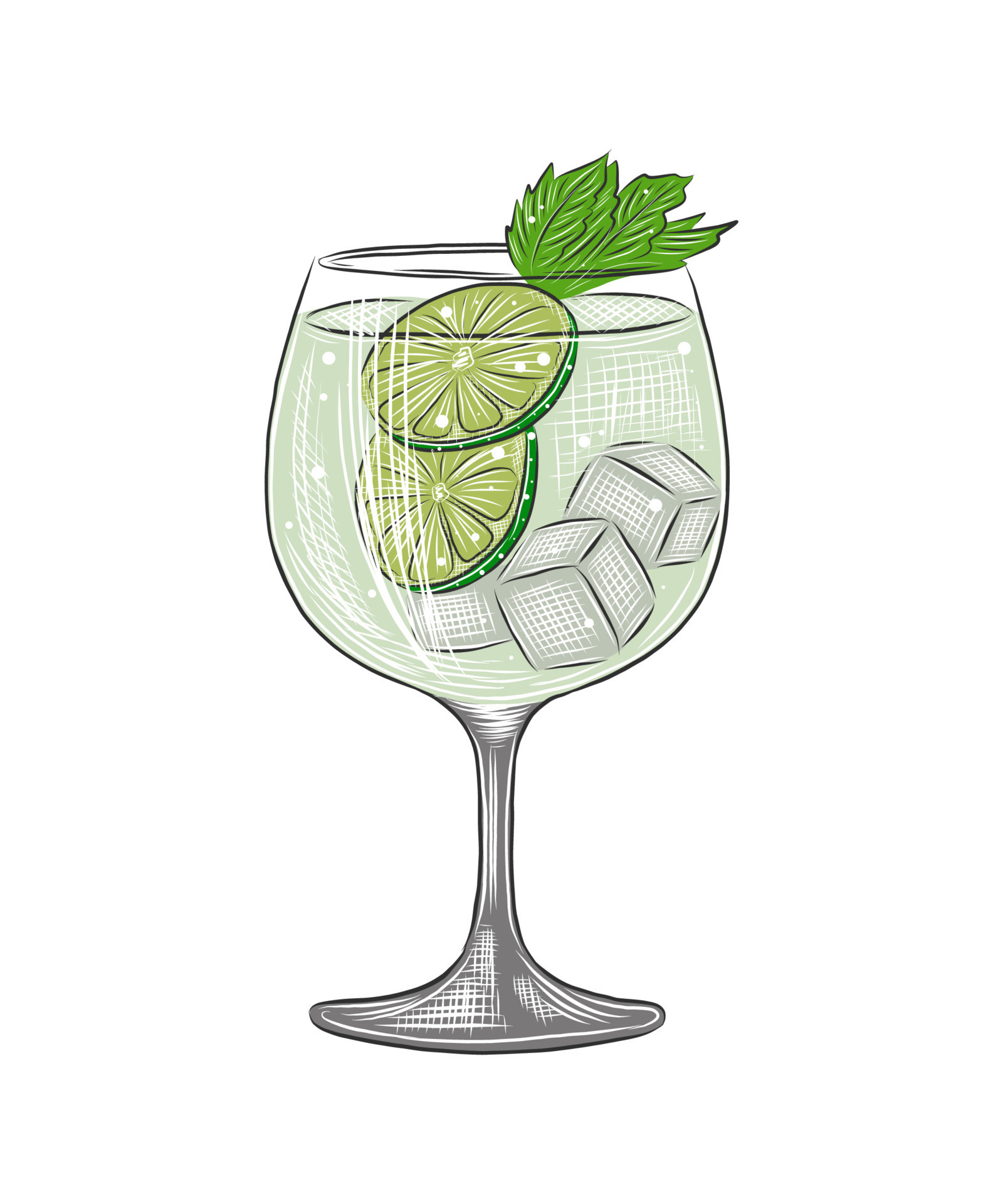The drawing depicts a glass filled with a light green liquid, likely a refreshing limeade. The glass resembles a wide-rimmed margarita glass, featuring a slender stem that extends down into a gray base. The liquid inside is accompanied by three cubical ice cubes, which are illustrated with gray and white checkered patterns. Adding to the refreshing appearance, two vibrant green lime slices float within the glass. A sprig of green mint extends out from the top of the liquid, providing a fresh garnish. The background of the image is white, emphasizing the detailed elements of the glass and its contents. The liquid contains small white circles, suggesting it might be carbonated, with effervescent bubbles rising through the beverage.